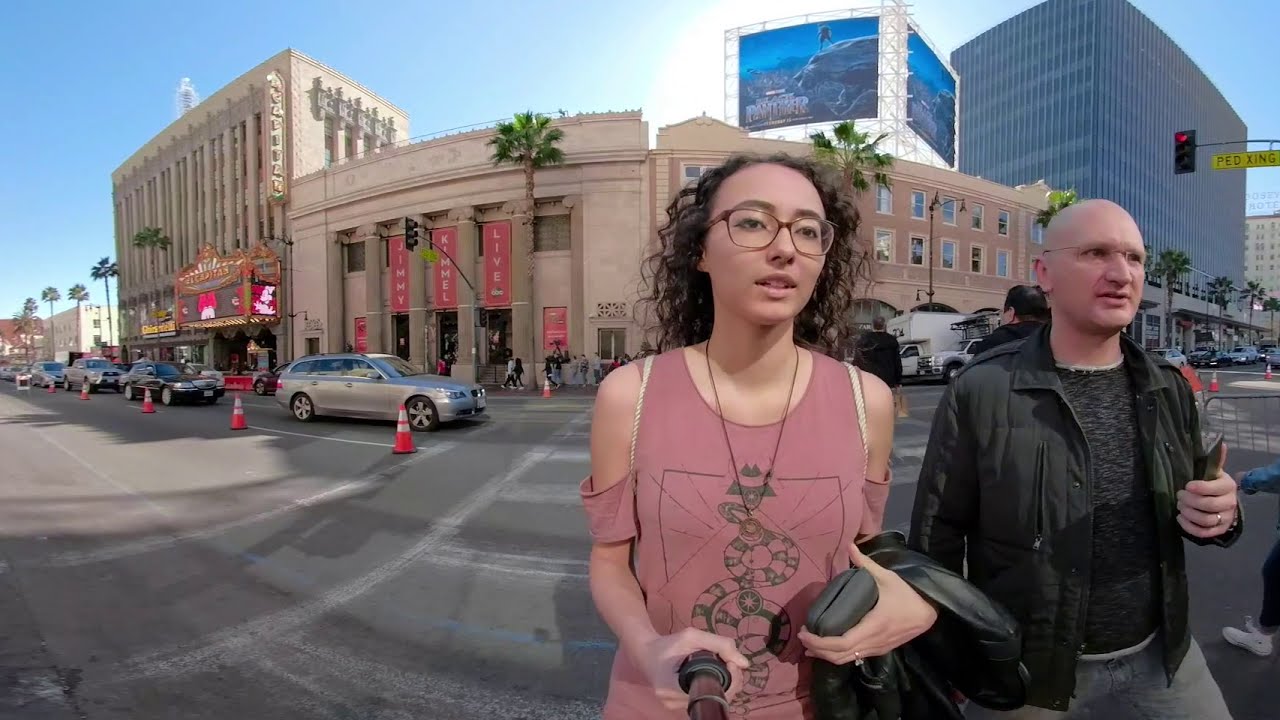In this vibrant cityscape photograph, a white woman with long, curly, brown hair, adorned in large square glasses and a pink tank top featuring a black snake design, stands just right of center. She holds a selfie stick in her left hand, capturing the moment, while her right hand clutches a clutch purse and perhaps a cell phone. A long leather cord necklace and a leather jacket draped over her right arm complement her stylish appearance, completed by a ring on her finger. Standing to her right is a bald white man, sporting glasses, a black zip-up jacket over a matching t-shirt, and a pair of blue jeans.

The duo appears to be in motion, crossing a city street, possibly in a place like LA, characterized by the presence of palm trees and bustling traffic. Behind them, a crosswalk intersects a busy street lined with cars. The backdrop includes notable buildings such as an older three-story theater to the right and a six-story office building to the left. The panoramic perspective captures their leisurely stride towards the bottom left corner of the frame, set against the lively urban scene.